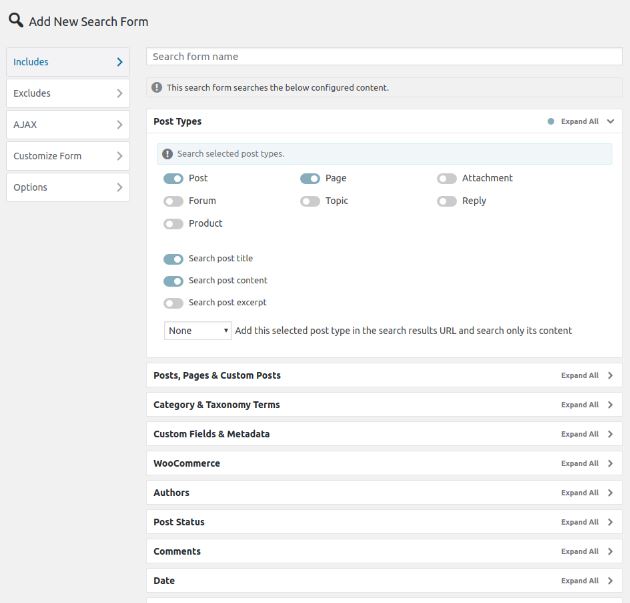This image showcases a "Add New Search Form" page, prominently displayed at the upper left-hand side, accompanied by a magnifying glass icon. The interface features a vertical menu on the left side of the screen. The menu items include "Includes," "Excludes," "Ajax," "Customized Form," and "Options." The "Includes" section is currently selected, revealing a box to the right-hand center.

Inside this box, there is a field titled "Search Form Name," with a white bar beneath it meant for input. Below this, there is a line of text stating, "This search form searches the below content types for you." Further down, options labeled "Post Types" can be seen, along with an "Expand All" button that has a drop-down arrow next to it.

Additional toggle options are listed underneath, with "Toggle Post," "Page," "Post," and "Search Post Titles" all turned on, as indicated by their "on" state. "Search Post Content" is also active. The image further displays a list of sample post, page, and custom post types at the bottom.

This detailed overview of the "Add New Search Form" page highlights its user interface and various functional elements.